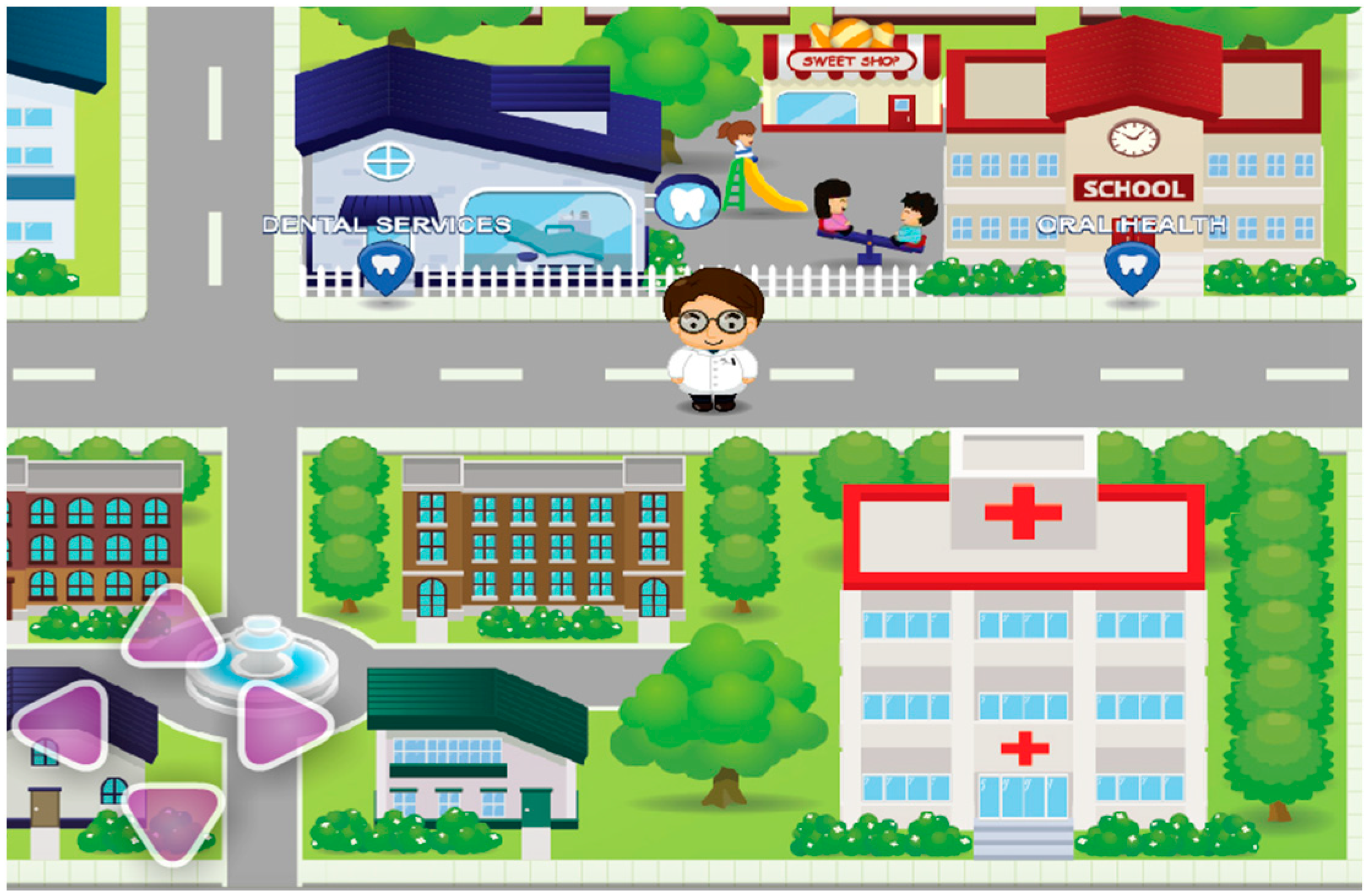The image is a simple, colorful cartoon depiction of a small city, resembling a screenshot from a children's computer or mobile game. At the center stands a doctor, likely a dentist, in front of a building labeled "Dental Services." To the right of this, there is a school named "Oral Health School," with children actively playing on a slide and a seesaw between the two buildings. Behind the children, a smaller sweet shop can be seen in the distance. In the upper right corner of the image sits the school, and in the lower right corner is a hospital marked with red crosses on top and above its doors. The cityscape includes trees scattered throughout and unmarked buildings, including a house in the upper left corner. The lower left features arrows resembling video game buttons, further suggesting the image is from a game. The scene has a playful, childlike quality, with elements that might appeal to young players.